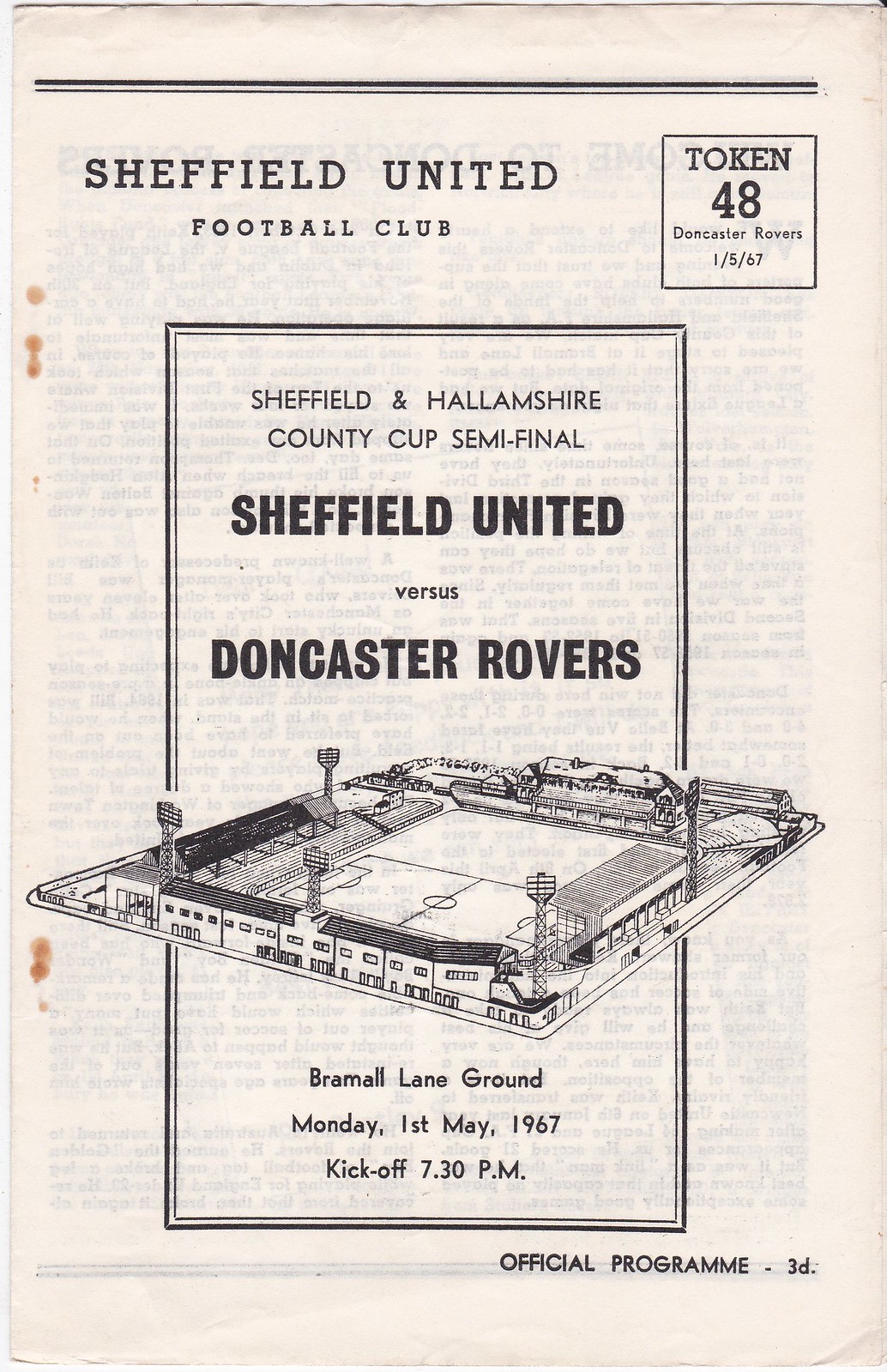This is a black and white official program cover from 1967, published by the Sheffield United Football Club for a match against Doncaster Rovers. The cover is notably simple and dated, with several brownish stains on the left-hand side, likely from spilled coffee or soda, indicative of its age. The paper itself is white and somewhat translucent, revealing shadows of the print from the other side. At the top left, the text reads "Sheffield United Football Club," with horizontal black lines above. There is a central, fairly detailed sketch of the Bramall Lane stadium, rather than a photograph. Below this, the text announces the Sheffield and Hallamshire County Cup Semi-Final: Sheffield United versus Doncaster Rovers, scheduled for Monday, 1st May 1967, with a kickoff at 7.30pm. Additional details include "Token 48" and the phrase "Official Program - 3D" in the lower right corner, all against a backdrop of aging yet well-preserved paper.